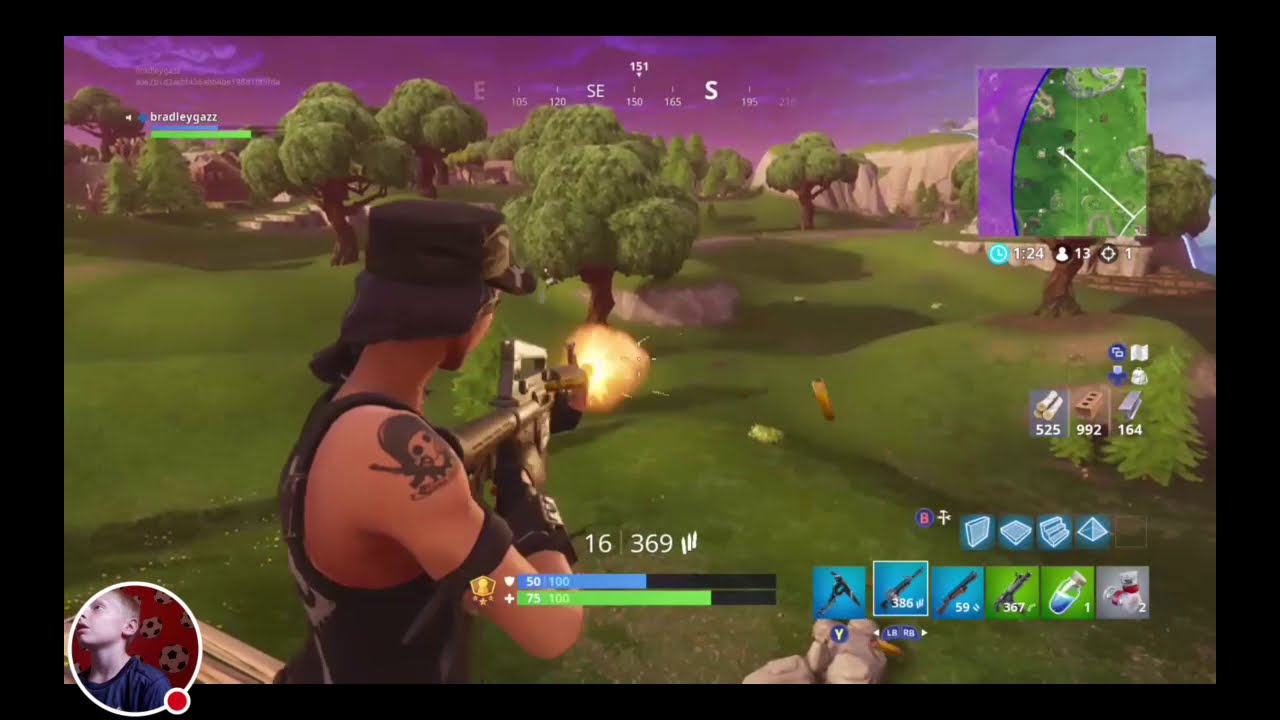The image depicts a vibrant and animated screenshot from a computer game. The scene is set within a horizontally rectangular frame bordered by a black edge. At the center of the action is a muscular figure, possibly a man, sporting a black tank top, a black cap, black gloves, and a skull tattoo on his arm. His hair is tied back into a ponytail at his neck. The character is holding a large rifle, from which fire and smoke emanate, indicating active shooting. Golden cartridge shells can be seen ejecting from the gun.

He stands on green grass, surrounded by cartoonish trees with large brown trunks and bushy green foliage, against a backdrop of rolling hills. Further in the distance, there are a couple of mountains and indistinct cartoon houses. The sky above is a vibrant mix of purple and blue hues, speckled with darker clouds. Near the character’s feet are a few stones.

In the lower right corner of the screen, a menu displaying various selectable items, including different guns, is visible. Additionally, a map is located in the upper right hand corner. In the lower left corner, a circular inset shows what appears to be a young Caucasian boy, possibly the player, with his face lit up as he gazes at the screen. He is seated in a room adorned with black wallpaper featuring soccer ball prints and is wearing a blue t-shirt. This detailed setup suggests an engaging and animated gaming experience with rich visual elements.